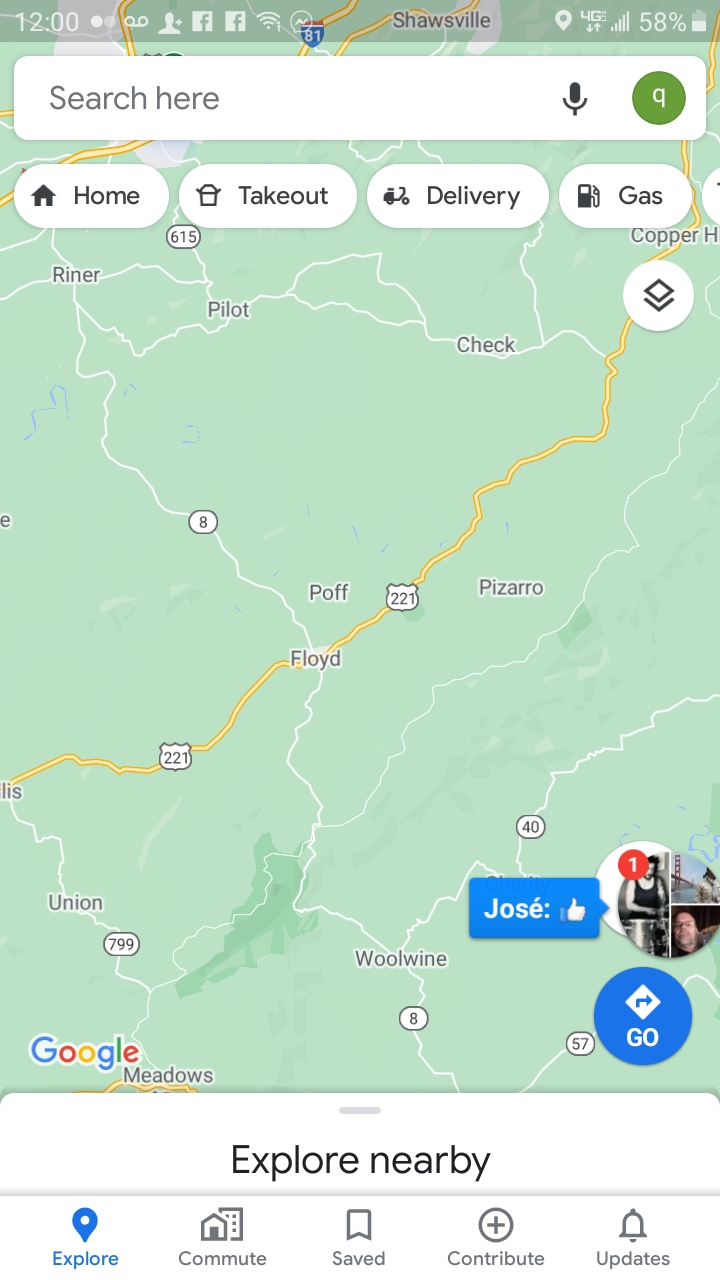This is a detailed screenshot of Google Maps displayed on a smartphone in light mode. At the very top, the phone’s notification bar shows it is 12 o'clock and contains several icons: a voicemail icon, a Google Hangouts icon featuring a man with a plus sign, two Facebook notifications, a Wi-Fi notification, and a battery status showing 58% remaining. Below the notification bar, there is a search bar labeled "Start search here," accompanied by a microphone icon and the profile icon of the user, depicted with an initial 'Q' in a green circle.

Adjacent to the search bar are quick access options including 'Home,' 'Takeout,' 'Delivery,' and 'Gas.' The map itself highlights specific areas namely Reiner, Pilot, Czech, Poff, Pizarro, Floyd, Union, and Worldwine, which are located along Highway 221, State Highway 8, 799, and 615. Directly below the map are navigation options such as 'Explore Nearby,' 'Explore Commute,' 'Saved,' 'Contribute,' and 'Updates.'

At the lower portion of the screen, there is a user-reviewed location, identified by the name 'Jose,' which features a thumbs-up icon and a small picture, presumably of Jose himself.